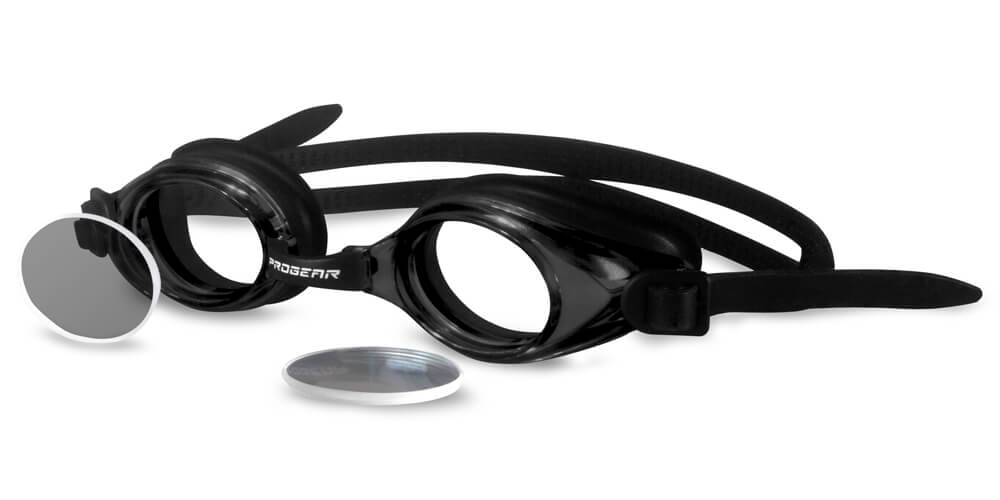This is a detailed photograph of black Progurph swimming goggles on a completely white background. The goggles feature clear, slightly tinted lenses, which are currently removed from the eye sockets; one lens is laying flat in front of the goggles, while the other is standing up at an angle. The goggles are designed with a black rubber strap and a black rubber frame, and the brand name "Proguph" is displayed in white text on the bridge connecting the two eye sockets. Additionally, the goggles come with protective snap-on caps for the lenses, which are also visible in the photograph. The image strictly focuses on the goggles and their accessories, with no other identifying information, such as price or store details, provided.